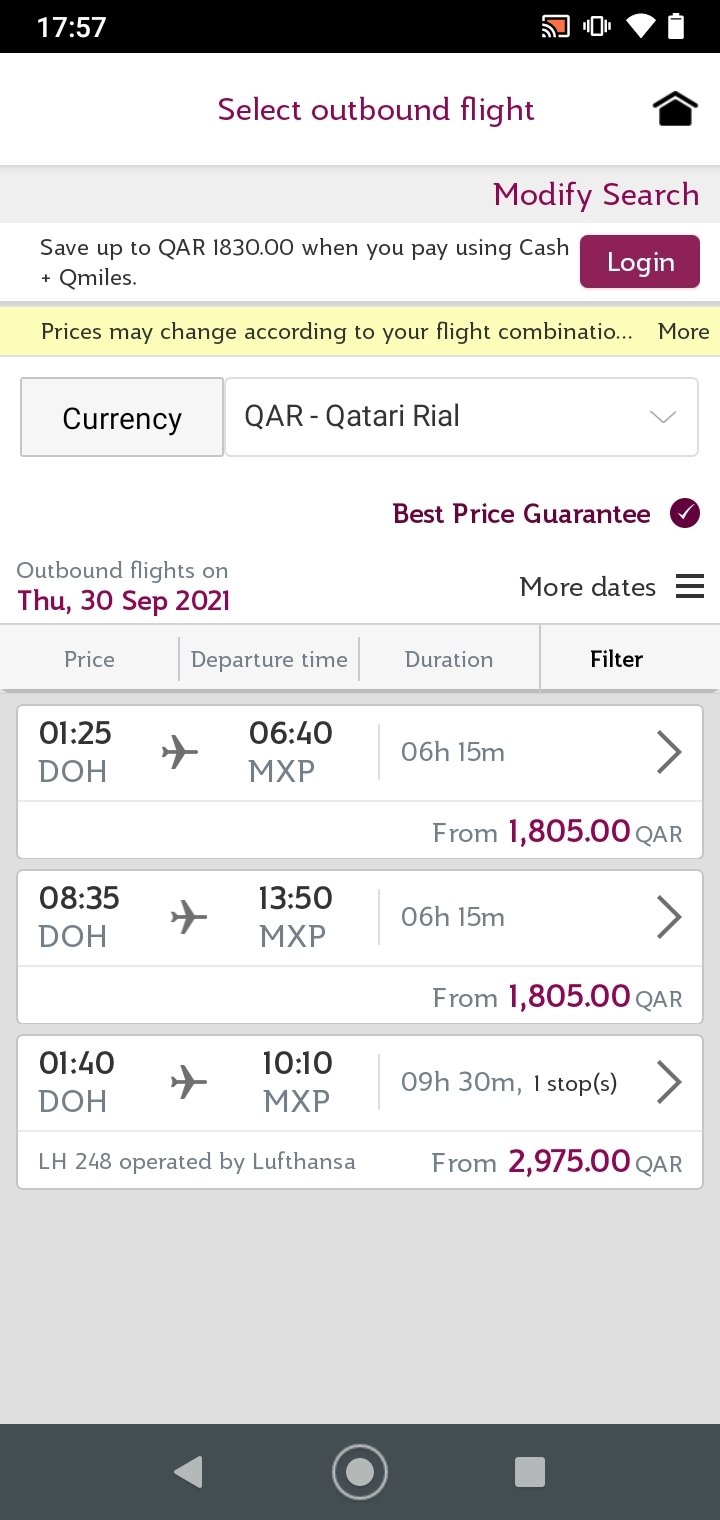The image portrays an iPhone screen displaying a flight booking app interface. At the top of the screen, in purple font, the text reads "Select Outbound Flight," accompanied by options to "Modify Search" and a message indicating savings of up to QAR 1830 when paying with Cash plus Qmiles. To the right of this saving message, the "Login" option is visible. 

Directly below this header, there is a horizontal yellow field with a cautionary note in black lettering: "Prices may change according to your flight combination." Immediately underneath, there is a currency button next to a field that indicates the selected currency as "QAR - Qatari Riyal."

Occupying the lower two-thirds of the screen, text assures "Best Price Guaranteed" for outbound flights scheduled on "THU, 30 SEP 2021." Below this assurance, a detailed grid displays flight information. Each row in the grid provides the flight details, including the departure and arrival times, duration, and price. 

The first listed flight departs at 12:40 PM from DOH (Doha) and arrives at 6:40 PM at MXP (Milan). The duration of this flight is specified as 6 hours and 15 minutes, with the price listed from 1805 QAR. Following rows in the matrix offer similar details for alternative flights with varying times but identical departure and destination airports. 

Overall, the interface is well-organized, displaying critical flight selection details in a structured format for the user's convenience.